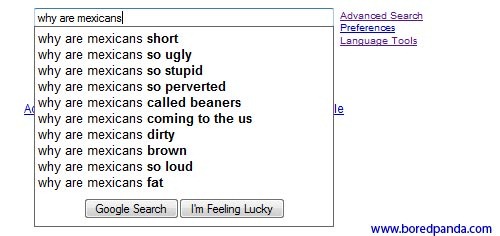The image is a screenshot of a Google search page, specifically capturing the autofill suggestions that appear when typing a query. The search input box at the top left contains the partially completed question, "why are Mexicans." The autocomplete results that follow exhibit derogatory and offensive stereotypes, listed as: "short," "so ugly," "so stupid," "so perverted," "called beaners," "coming to the US," "dirty," "brown," "so loud," and "fat." 

Below the search box, two buttons are visible: "Google Search" on the left and "I'm Feeling Lucky" on the right. To the right of the search box, additional links labeled "Advanced search," "Preferences," and "Language tools" are noted, providing ancillary navigation options. At the bottom of the screenshot, a link to "boredpanda.com" is visible, indicating the possible source of the image or additional related content. 

The image highlights the unsettling nature of some autocomplete predictions, shedding light on the prevalence of negative stereotypes in online search queries.